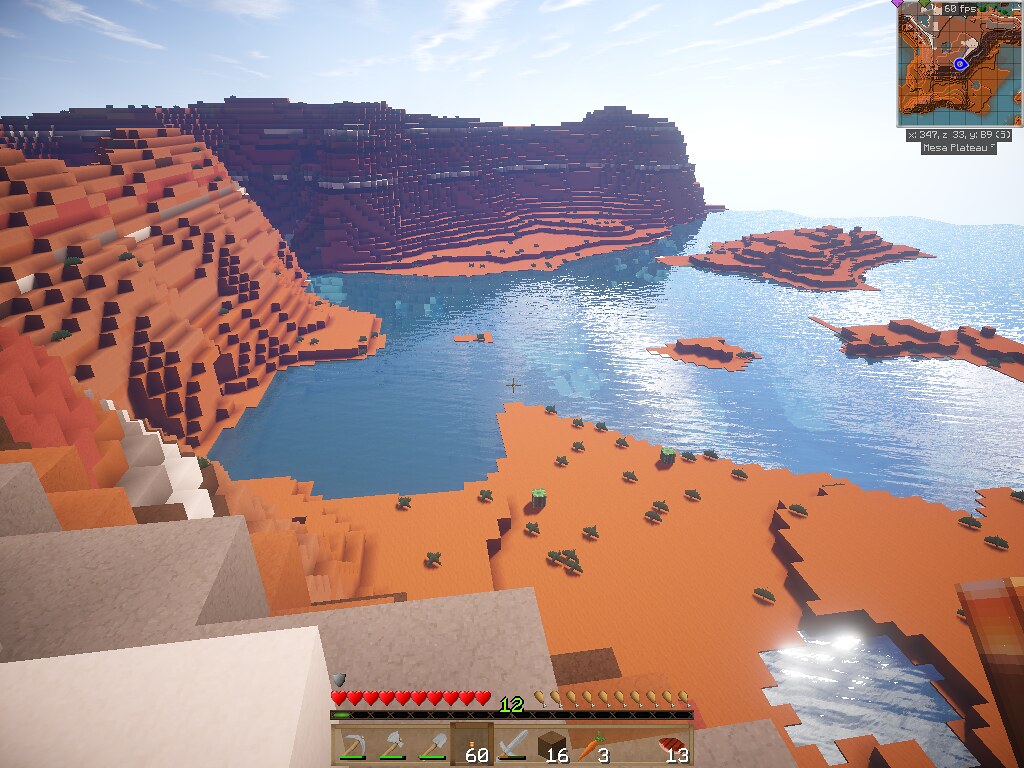This image is a detailed screenshot from a video game, most likely Minecraft, judging by the pixelated, blocky design and familiar interface elements. The scene depicts an expansive coastal landscape with a prominent view of various natural formations and a user interface overlay. The sky is a gradient of medium to light blue, scattered with thin white clouds. The foreground showcases a variety of sandy structures resembling cliffs and walls that partially enclose a body of water. To the left, a large light brown cliff juts into the ocean, while towards the center, there are darker hills and additional cliffs. Numerous small, roundish islands can be seen dotted across the water, with their elevated parts shaded in darker hues. In the upper right corner, a mini-map displays the surrounding area, indicating the player's position. Below the scene, the game interface is visible, displaying a row of hearts for health, a row of chicken legs presumably representing hunger, and some boxed tools. There is also a numerical indicator showing "12" in green between the hearts and chicken legs.